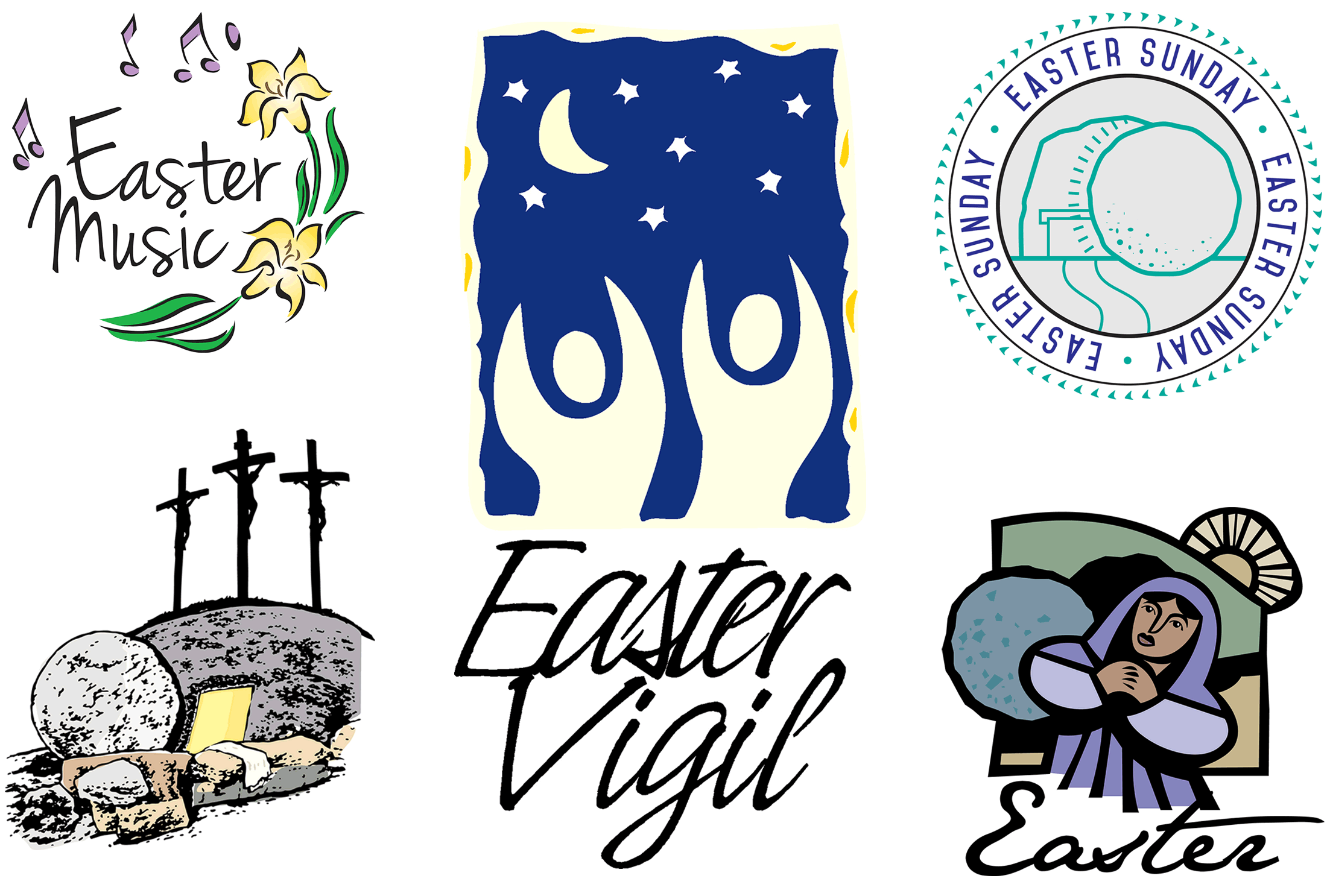This image set comprises various detailed graphic designs celebrating Easter, possibly for a church event or service. In the upper left-hand corner, there's a graphic titled "Easter Music" in black cursive, featuring yellow tulips and purple musical notes. The upper middle image shows two white silhouettes with their hands raised towards a night sky filled with stars and a crescent moon on a deep blue background. Below them, "Easter Vigil" is written in black cursive. The upper right image is a circular design with the words "Easter Sunday" in blue uppercase letters, repeated in a ring around a central depiction of a cave with the stone rolled away, symbolizing the resurrection. In the bottom left, there's a gray illustration of a cave with a glowing interior, topped with three crosses, representing Jesus's crucifixion and resurrection. The bottom middle image also says "Easter Vigil" in cursive, tying into the central theme of nighttime celebration. Finally, in the bottom right, there is a stylized graphic of a woman, possibly representing Mary Magdalene, in a purple dress and hood, praying in front of an open cave with a stone rolled away, and the word "Easter" in bold cursive above her.